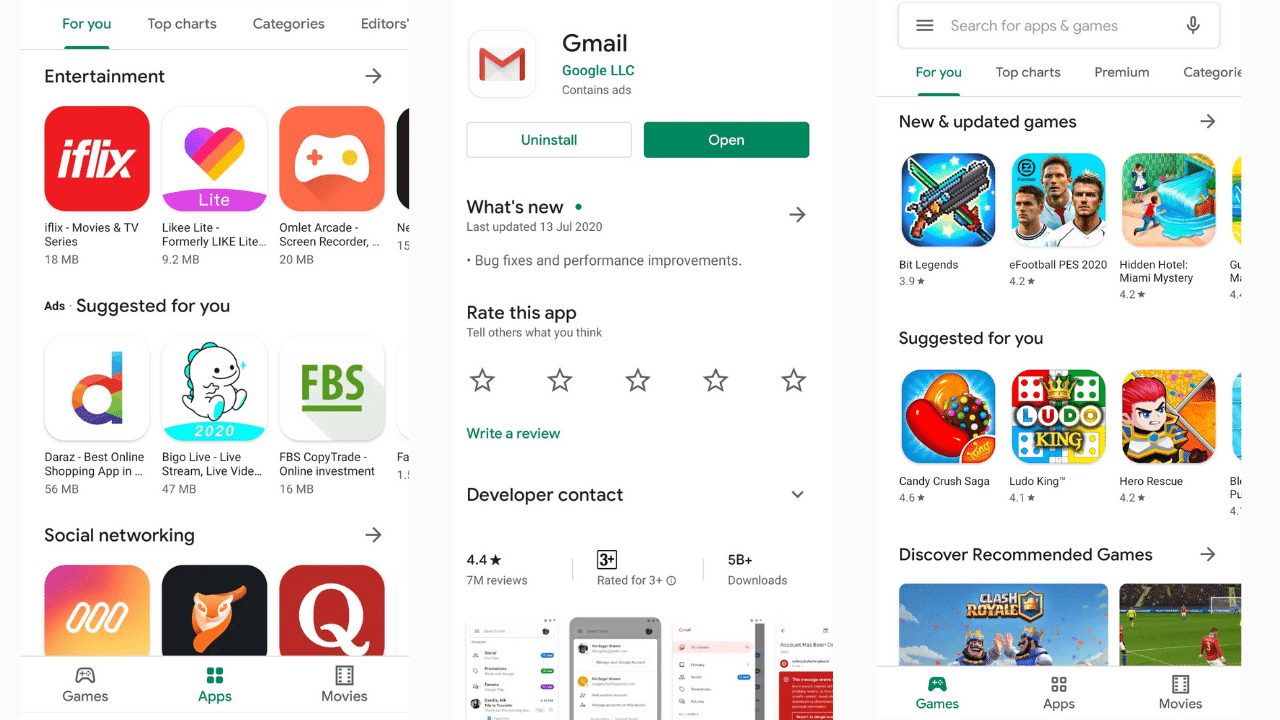The image contains three screenshots from an app store interface. 

- The leftmost screenshot is under the "For You" tab, displaying various app categories such as "Entertainment" and "Social Networking," along with a section titled "Suggested for You."

- The middle screenshot showcases the Gmail app. This view includes a green "Open" button on the right and a white "Uninstall" button on the left. Below, there are sections labeled "What's New," "Rate This App," and "Developer Contact."

- The rightmost screenshot features several app categories under the "For You" section, including "New and Updated Games," "Suggested for You," and "Discover Recommended Games." At the bottom of this screenshot, there are three icons labeled "Games," "Apps," and "Movies."

The images collectively display a range of personalized app recommendations and various navigation options available in the app store.